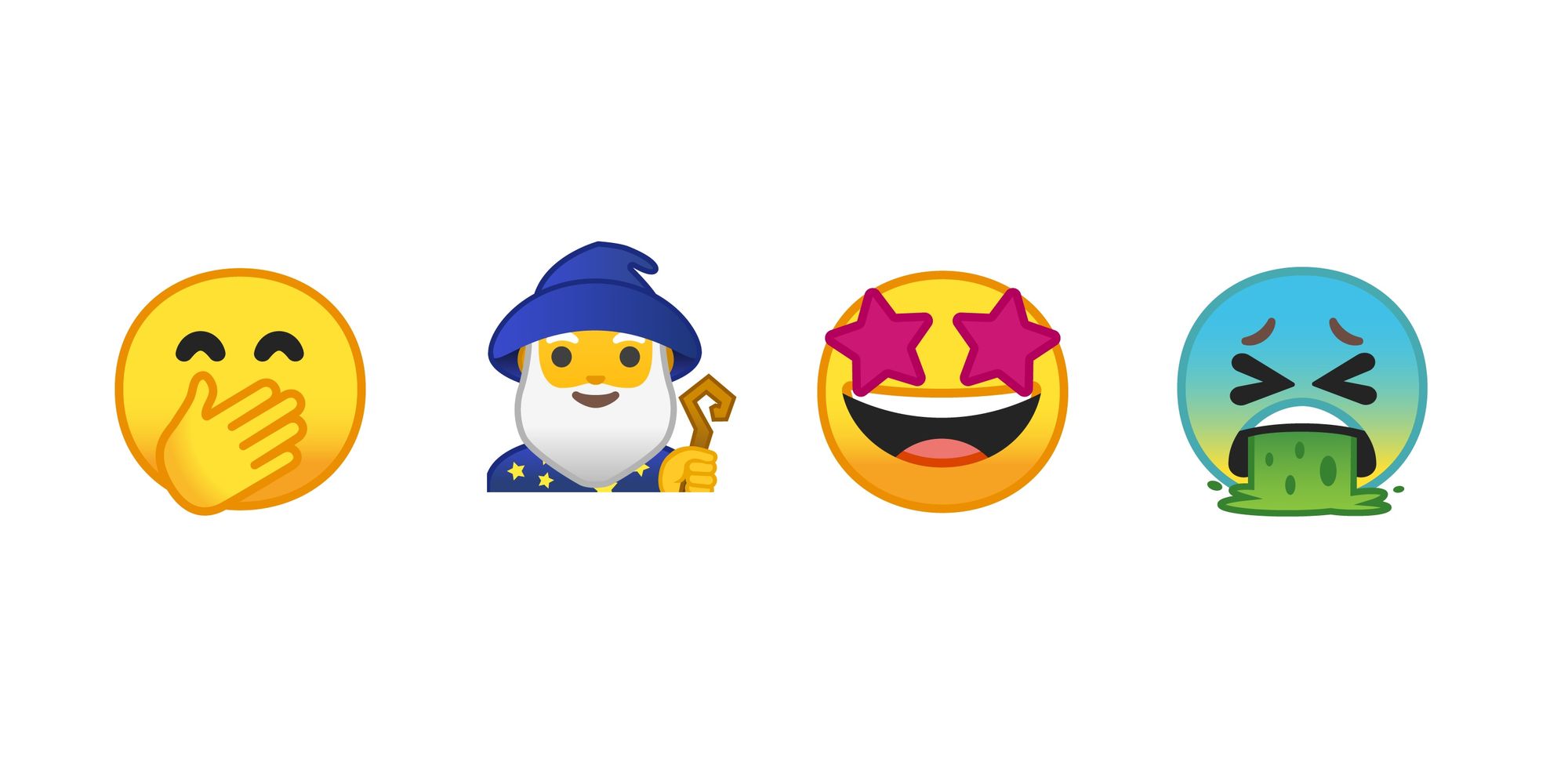This image features a collection of four emojis on a plain white background, each exhibiting a distinct character and expression. The emoji on the far left is a coy smiley with its right hand covering its mouth, eyes closed as if giggling or reacting bashfully. Next is a wizard emoji, characterized by a long white beard, a blue cloak adorned with gold stars, a matching wizard hat, and a wooden staff in his left hand. The third emoji showcases a starstruck face, its eyes replaced by deep magenta stars, and a wide, excited smile. Finally, the emoji on the far right depicts a sick face, colored teal with tightly shut eyes, and spewing green vomit. Although they are recognizable, these emojis appear to be custom or platform-specific variations, slightly recolored or tweaked versions of standard emojis.